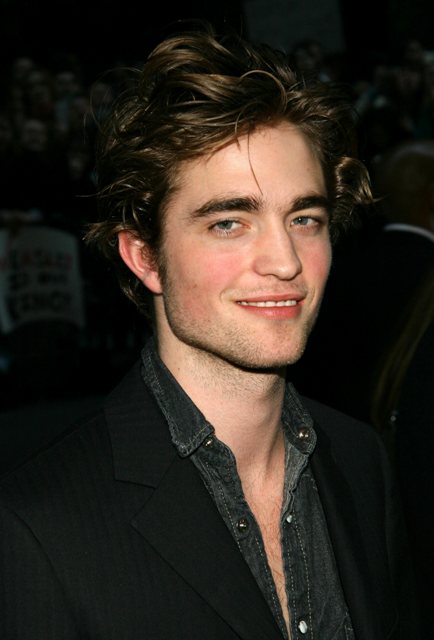The photograph features a young man, likely in his early twenties, with delicate facial features and slightly rosy cheeks. He has blue eyes, dark bushy eyebrows, and unshaven face. His brown, wavy hair is styled to swoop up and away from the center, giving it a somewhat tousled look. He wears a dark, denim-like shirt, perhaps a snap-up or button-up style, which is partially unbuttoned to reveal a hint of chest hair. Over this shirt, he is clad in a black blazer with thin gray lines and noticeable silvery buttons. He sports a subtle, welcoming smile, showing his white teeth. The background is very dark and blurred, with indistinct shapes that could be a crowd of people or chairs, but the details remain unclear. The overall atmosphere suggests he might be at an event or personal appearance.